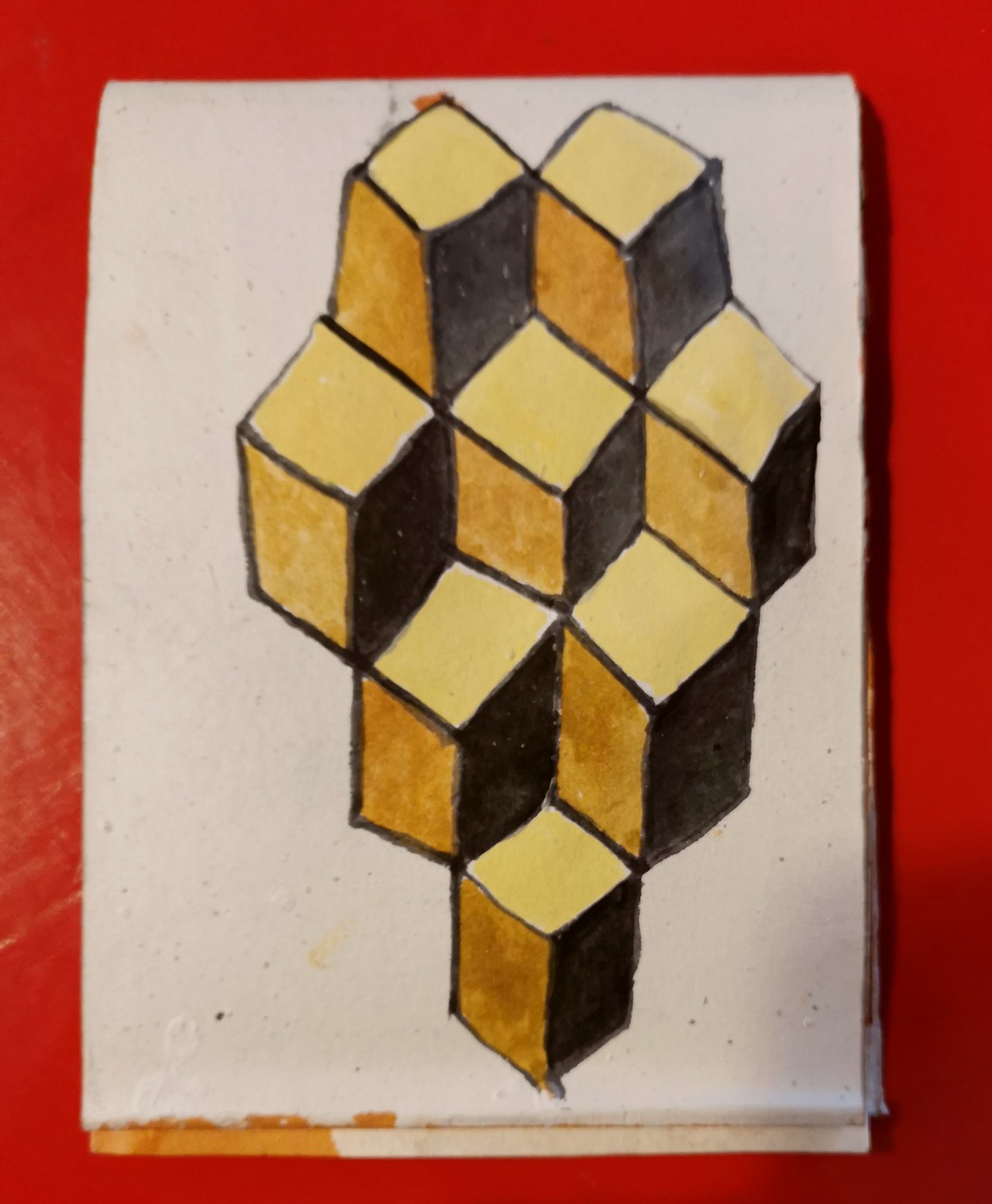A detailed painting on what appears to be homemade, speckled, off-white paper, set against a bold red background. The textured paper, either placed on a red table or fixed to a red wall, creates a striking contrast with the artwork it holds. The painting features a collection of geometric cubes, rendered in varying shades of golden yellow. The tops of the cubes are highlighted with a brighter yellow, while the right sides are shaded in black, giving them a three-dimensional appearance. The cubes are meticulously arranged in a honeycomb-like structure, though maintaining their cube shapes. Visible are eight individual cubes, but the overall geometric formation suggests a larger, interconnected structure that invites consideration of mathematical principles. The entire composition is slightly off-center, skewed towards the right side of the paper, adding a dynamic element to the piece.